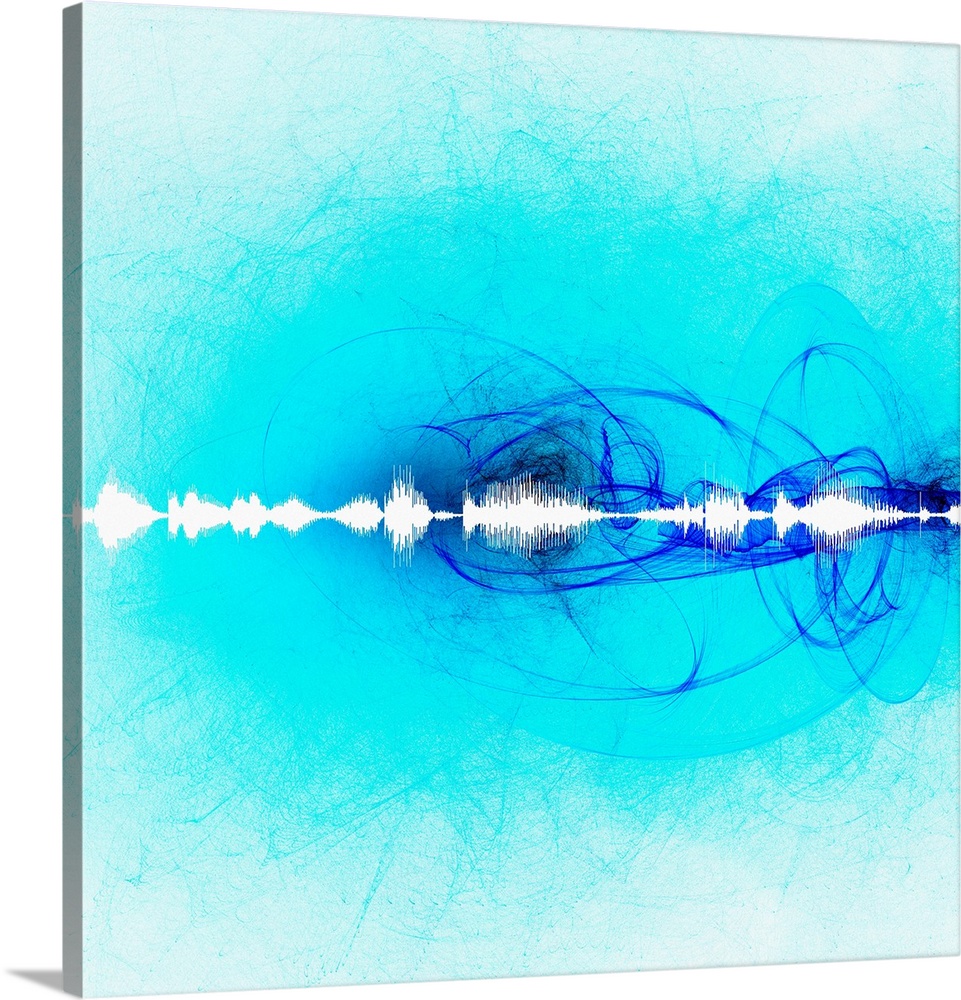This image features a modern art piece displayed on a square, thin canvas with light blue and teal hues. The canvas, depicted at an angle with sides barely visible, casts a subtle shadow on the bottom right against a transparent background, giving it a slight 3D effect. Central to the composition is an irregular white sound wave running horizontally across the middle, its peaks and troughs varying in size and shape. Beneath this waveform, the background shifts from light smudged blue to vibrant teal, with deep blue swirls and geometric wisps accentuating the abstract design. The overall texture reveals thin brush strokes across the canvas, adding to the detailed and dynamic visual appeal.